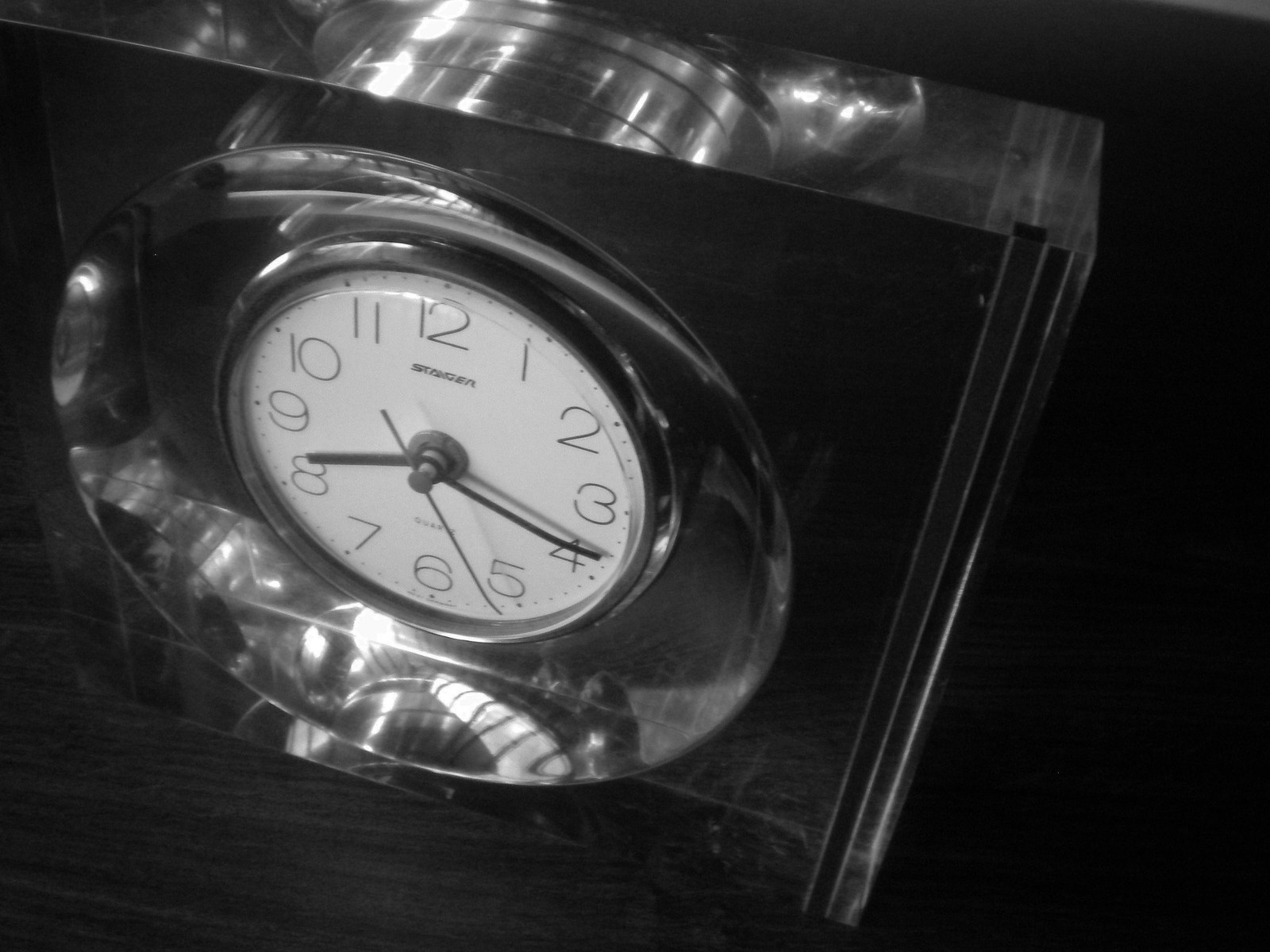This black and white photo captures a close-up of an analog clock with a white face, featuring regular numbers 1 through 12 in English. The clock displays the time as 8:19 and 27 seconds with black metal hour, minute, and second hands. Enclosed within a clear, crystal-like plastic block, the clock has a silver band around its face. The block features a cutout, adding depth to the image and creating reflections that catch the ambient light and the back of the clock at the top of the photo. The clock and its crystal case are set against a dark background, possibly a very dark wood table. An unreadable word appears near the number 12, adding a subtle detail to the image’s composition.